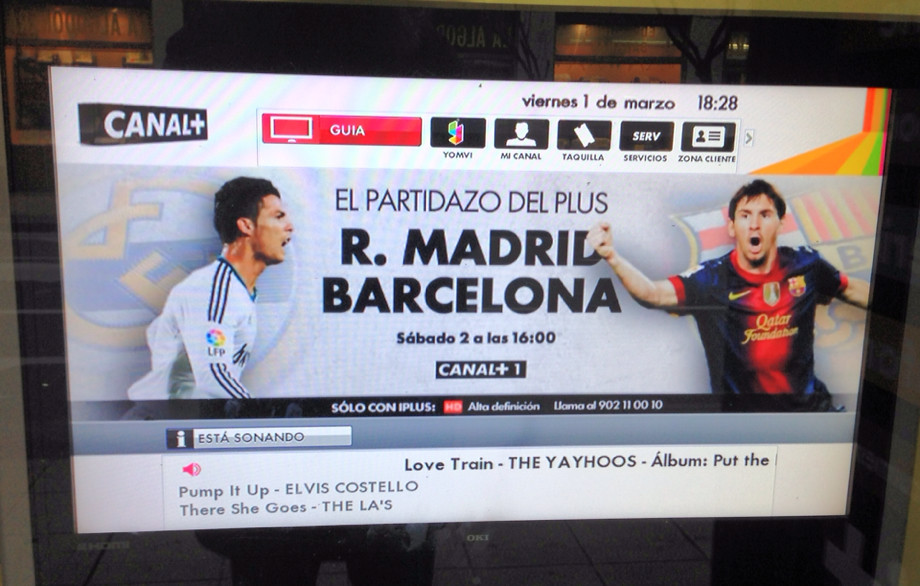This is an advertisement for an upcoming football match between Real Madrid and Barcelona, shown as a glossy photograph of a television screen. The ad, primarily in Spanish, features two athletes in their team uniforms—one in dark blue and red, the other in white with blue stripes. The backdrop displays the logos of the respective teams, with a noticeable logo in a black box reading "Canal Plus” on the upper left, accompanied by menu options where the selected item is highlighted in red. The date and time are prominently displayed: "Viernes 1 de Marzo 18:28" (Friday, March 1, 18:28) at the top, and "Sábado 2 a las 1600" (Saturday at 16:00) in the center, alongside the match title "El Partidazo del Plus" and the teams "R. Madrid" and "Barcelona." Below the central graphic, there is music information, mentioning the current song "Love Train" by The Yayahus and upcoming tracks including "Pump It Up" by Elvis Costello and "There She Goes" by The L.A.'s. The main colors in the image are white, black, blue, and red, enhancing the vivid visual presentation of this high-stakes sporting event.